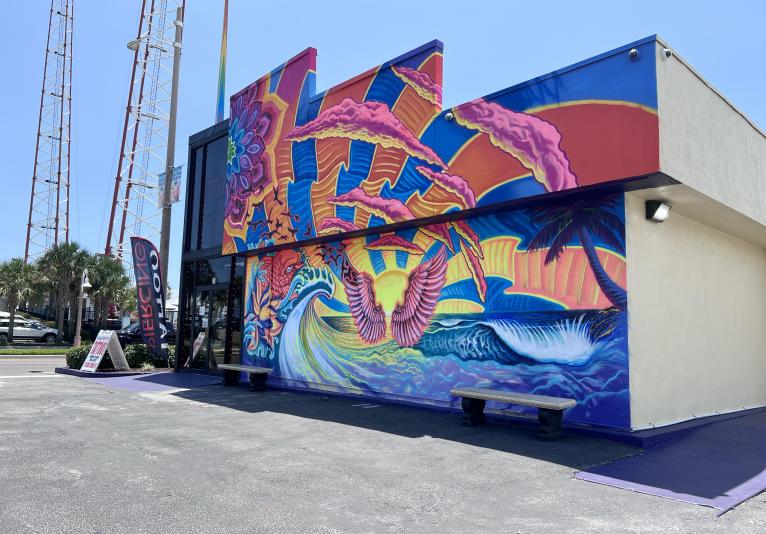The image captures a vibrant outdoor scene featuring the side of a small building on a sunny day. Dominating the view is a striking mural on the front wall of the building, which is sectioned into two halves. The mural artistically depicts dramatic blue sea waves at the bottom, interspersed with abstract elements like a pink bird on the left and splashes of yellow and pink throughout. Above the waves, the upper section showcases a radiant sunset with wavy rays in orange and yellow, twisting upwards and outlined in red. Surrounding the sun are ethereal pink wings. There's a whimsical combination of purple flowers, purple and orange lines, and purple clouds distributed in the middle and right side of the mural. A blue palm tree branches into the scene from the upper right, adding a splash of cool color.

Adjacent to the mural, on the left, a section of the building features a large glass window outlined in black with a door at the bottom and a big window above it. In the distance beyond this window, two metal towers, likely cell phone towers, extend out of the frame. The scene is grounded by a simple, gray concrete area in front of the building, where two benches and a security light are also visible. Farther in the distance, a parking lot, complete with a white truck, is partially visible, emphasizing the building's urban setting.